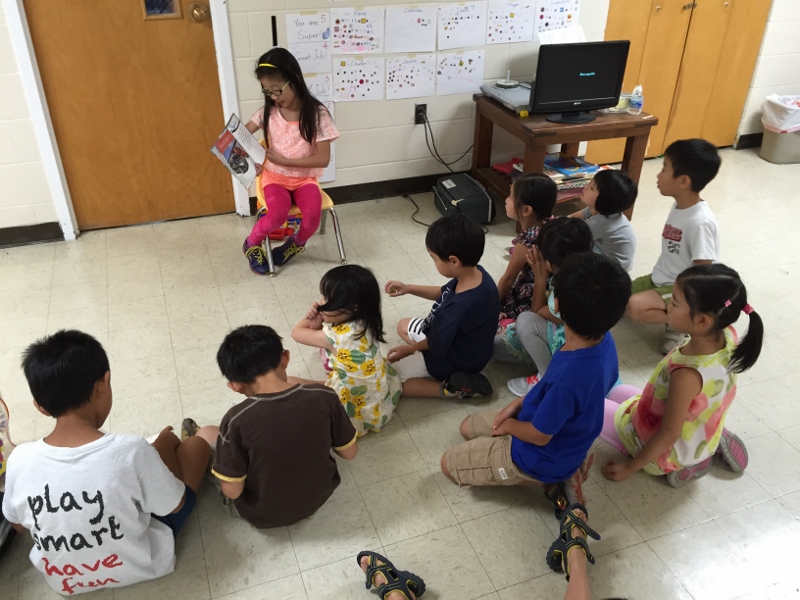A horizontal rectangular photograph captures a lively elementary school classroom scene, featuring a young girl with long dark hair and dark skin sitting in a child-sized yellow chair at the front. She is wearing an orange top and red pants, reading a book or magazine to her classmates. The classroom is filled with at least 10 children ranging in age from 3 to 7, seated on a white linoleum floor, with some sitting on their bottoms and others on their knees. The children, dressed in various bright colors, are scattered on the floor, fidgeting and showing varying levels of attention to the reader. Notable classroom details include self-drawn artwork on the walls, a plugged-in monitor, a brown door, and a closet. The atmosphere suggests a typical spring day in a diverse and vibrant educational setting.